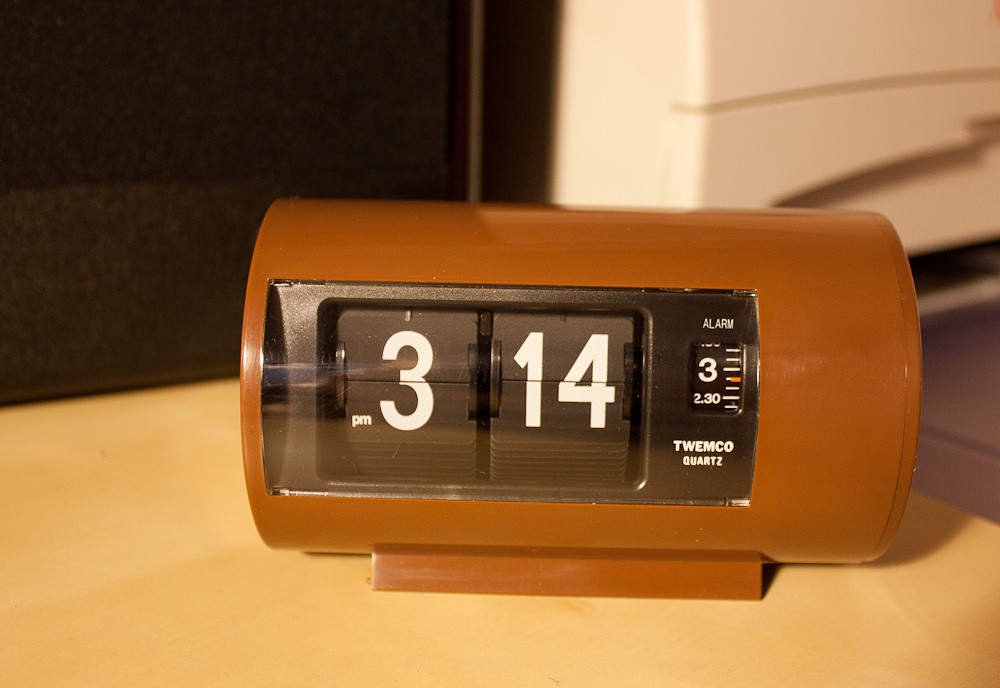The photograph captures a vintage-style alarm clock with a cylindrical body, finished in a rich dark brown color. The central area of the cylinder features a rectangular display, where the time is indicated. This display showcases a black plastic background contrasted by two smaller black squares designed to flip and reveal the time. On the left square, "P.M. 3" is displayed in clear white text, while the right square shows "14". Above the right square, in smaller white text, the word "alarm" is inscribed. Below this, there is a mechanism to set the alarm, and just beneath that, the brand name "Twimco Quartz" is clearly written in white. The clock is placed on a light tan table or desk, adding a nostalgic element to the setting.